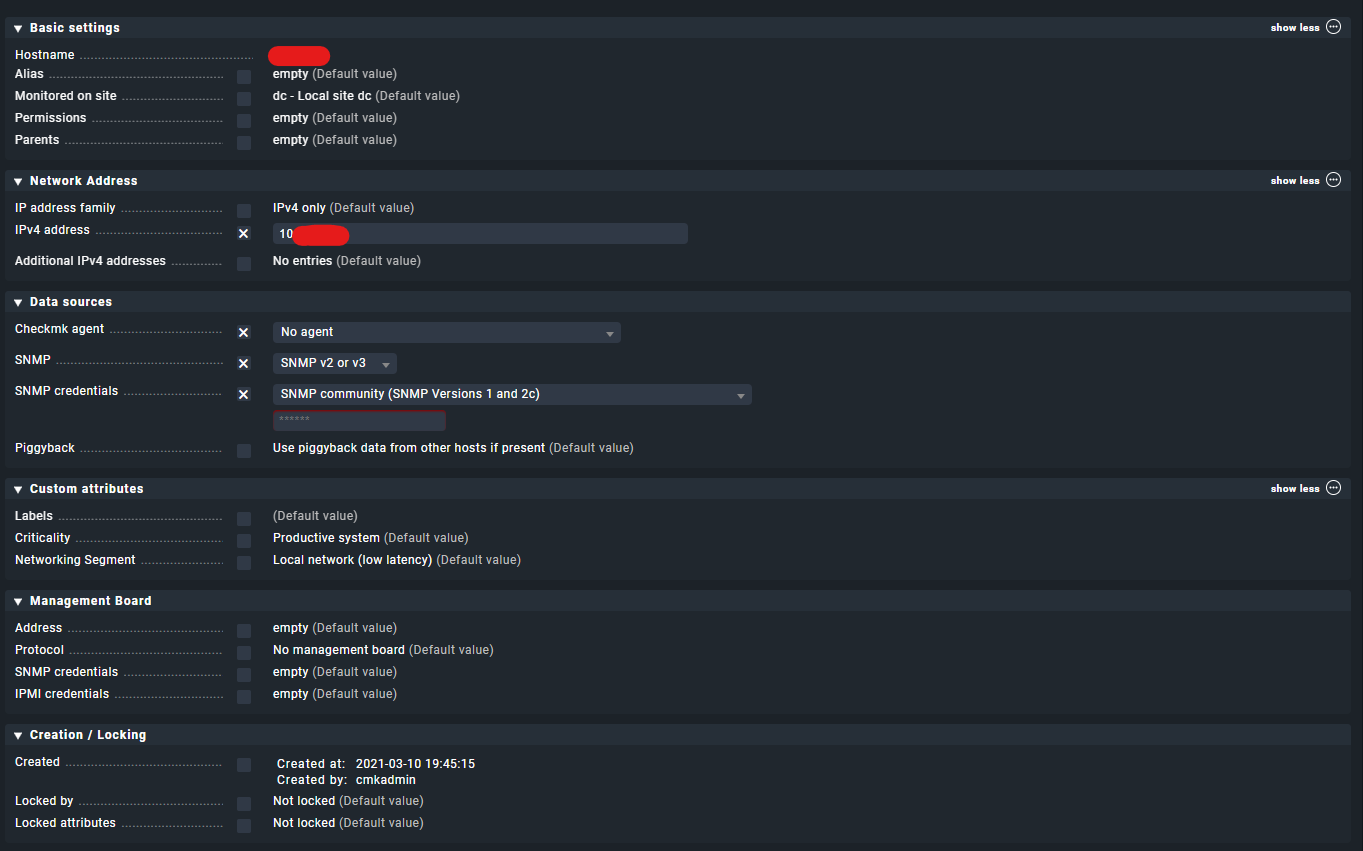In the upper section of the interface, "Basic Settings" is prominently displayed. To the right, there is a red box obscuring some content, with adjacent text indicating "Empty Default Value," "Local Site DC Default Value," followed by repeated mentions of "Empty Default Value." 

Below this, it specifies "IPv4 Only Default Value." Adjacent to this is another red oblong box covering additional content. Directly beneath, the phrase "No Entry Default Value" is visible, alongside a drop-down menu labeled "No Agent." Another drop-down menu offers the options "SNMP v2" or "SNMP v3."

Further down, the interface displays "SNMP Community," followed by "SNMP Version 1 and 2." Below this, there's an option labeled "Use Piggyback Data From Other Hosts," currently set to its "Present Default Value." Lastly, the interface mentions "Default Value" again and notes "Production System."